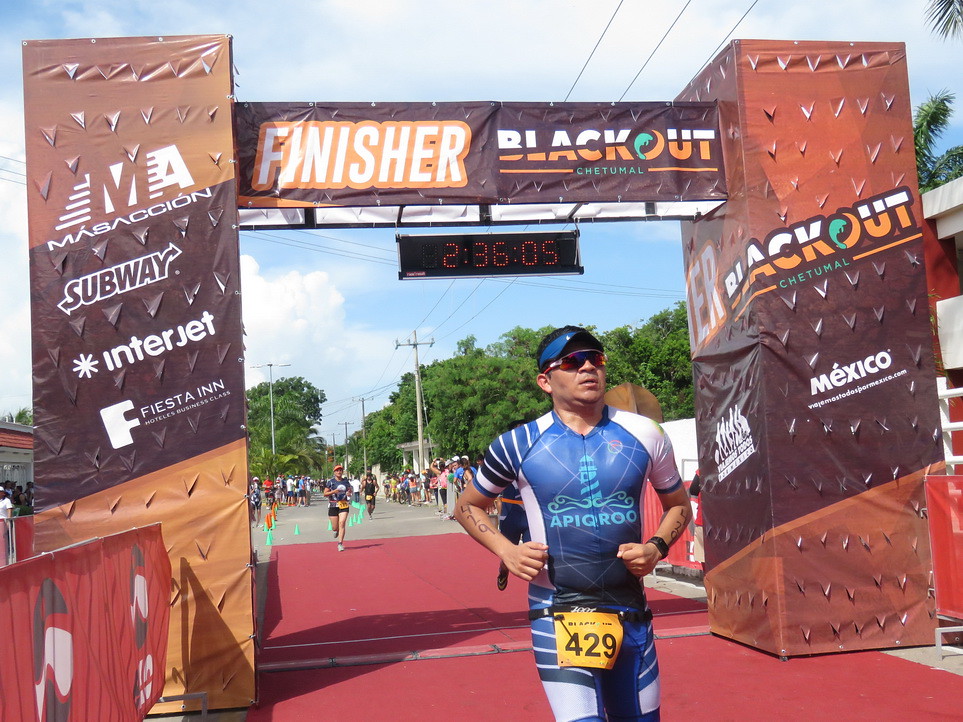In the photograph, a male runner, prominently positioned near the front, is captured crossing under a squared-off archway that signifies the race's finish line. The runner, wearing a blue and white bodysuit branded with "Epic Crew" and donning a blue visor along with red sunglasses, sports the number 429 displayed on a yellow sign strapped to his waist and also marked on his arms. The ground beneath him is covered with a red carpet leading up to the finish. Above him, the timer suspended from the archway displays a time of 2 hours, 36 minutes, and 5 seconds. The archway is adorned with various banners and advertisements, including brands like Subway, Interjet, Blackout, Fiesta Inn, Chetumal, and Mexico. Behind the runner, more participants are visible in the distance, approaching the finish line, while spectators stand behind barriers, watching the event unfold. This scene unfolds outdoors in daylight, capturing the concluding moments of the race.